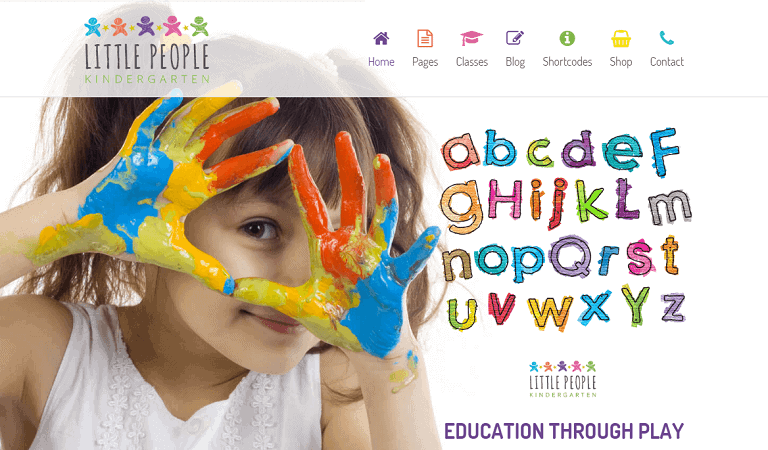The screenshot features a vibrant website titled "Little People." The homepage showcases a beautifully designed banner with the words "Little People" in various bright colors, reminiscent of watercolor art. At the center of this banner is an image of an adorable little girl with brown eyes and pigtails, curiously gazing at the viewer while holding her finger to her cheek. Her hands are smeared with colorful paint, indicating a playful and creative activity. She is dressed in a simple white top. Below the banner, navigation options are listed in watercolor-style text, including sections such as Homepages, Classes, Blogs, Shortcodes, Shop, and Contact. The "Little People" brand is prominently emphasized throughout the screenshot, reinforcing the educational and playful nature of the website.